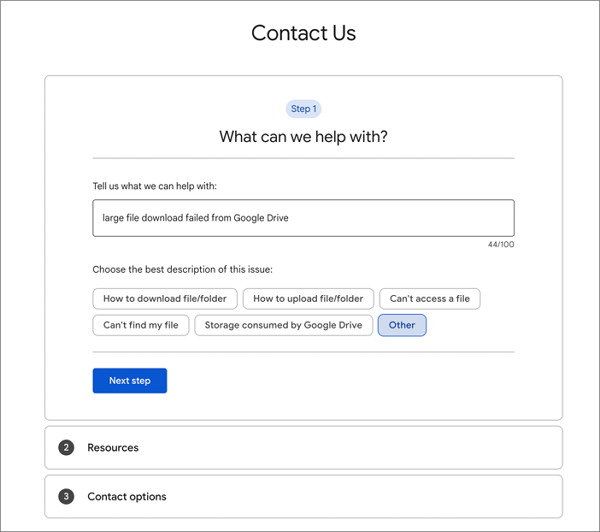This image depicts a contact page from a website designed for user inquiries. The page features a user-friendly form against a pristine white background. The form is enclosed within a thin black border, emphasizing its structure. At the top center of the form, bold black letters prominently display the heading "Contact Us."

Inside this outer box is another box with light gray, rounded borders, enhancing the visual appeal and organization. This inner section belongs to "Step One," indicated by a blue bubble at the top. This step is titled "What can we help with?" inviting users to describe their issue or inquiry.

Beneath this prompt, a text box is filled with the message: "Large file download failed from Google Drive," which uses 44 out of the 100 available characters. The form further asks the user to choose the best description of the issue from several options, including: "How to download file/folder," "How to upload file/folder," "Can't access a file," "Can't find my file," "Storage consumed by Google Drive," or "Other." In this instance, the option "Other" is selected.

At the bottom, there's a "Next Step" button leading to subsequent sections: "Step Two" and "Step Three," which likely comprise resource suggestions and contact options to assist the user further.